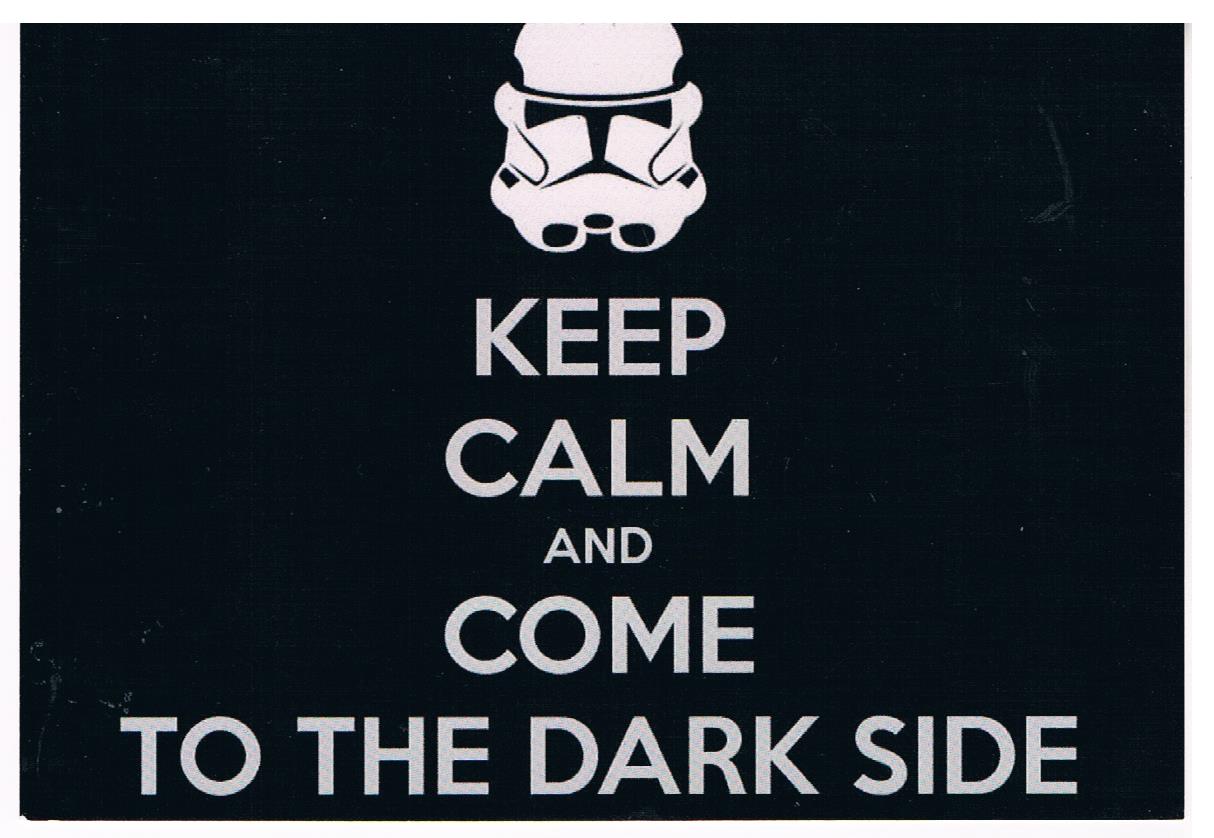This image features a rectangular black background adorned with subtle distress marks, most notably in the lower left and upper right corners. Faint scratches and white dots further contribute to the worn appearance. Dominating the top portion of the image is an illustrated outline of a white stormtrooper helmet from the Star Wars franchise. Beneath this helmet, bold, white, all-capital text reads "KEEP CALM AND COME TO THE DARK SIDE." The lack of additional context makes it unclear whether this design is from a poster, postcard, or another medium.